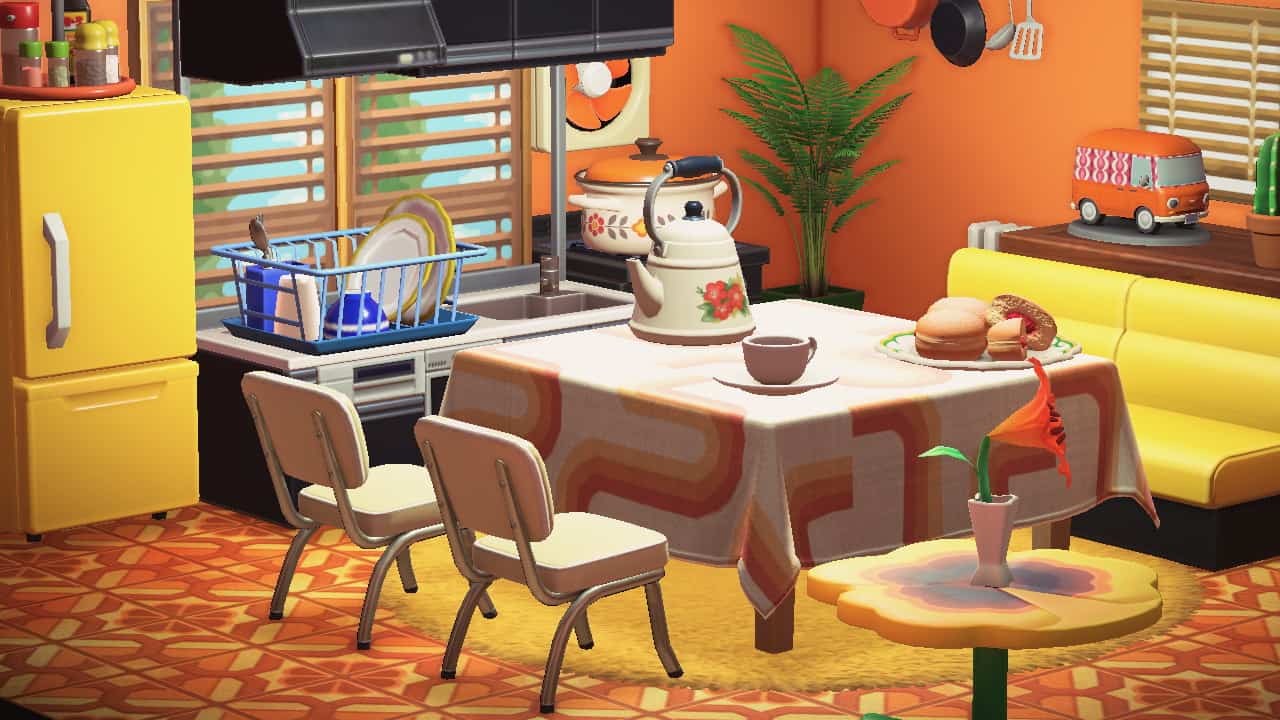The image depicts an AI-generated rendering of a kitchen with a distinct 60s-80s retro cartoonish style, characterized by vibrant, clumsy aesthetics. Dominating the room are bright orange walls and a mix of yellow and orange flooring. 

At the center stands a large table draped in a beige-pink tablecloth with red and orange stripes, atop which sit sizable cheeseburgers, donuts, a coffee cup, and a teapot that appears nearly as big as the table itself. Surrounding the table is a yellow rug, matching the room’s bold palette. Adjacent to the table is a yellow cushioned booth that resembles a couch, laden with orange and white linens.

To the left of the table is a yellow refrigerator, complete with a white handle, a top door, and a bottom drawer, with black wheels visible underneath. A red tray with spices rests on top of it. Directly next to the fridge are a sink and a stovetop, equipped with a blue strainer basket for drying dishes and a significant pot on the stove. Above the sink is a two-pane window with brown blinds pulled up, revealing a clear blue sky and two trees outside.

The kitchen also features 1950s-inspired metal chairs with pink cushions, contrasting with a red cushioned booth chair on the other side of the table. Decorative elements include a small flower vase on a side table, an orange bus-shaped ornament on a brown countertop, and a green palm tree situated between the stove, sink, and booth. The room's overall aesthetic is bright and colorful, merging nostalgia with a playful, almost surreal appearance.